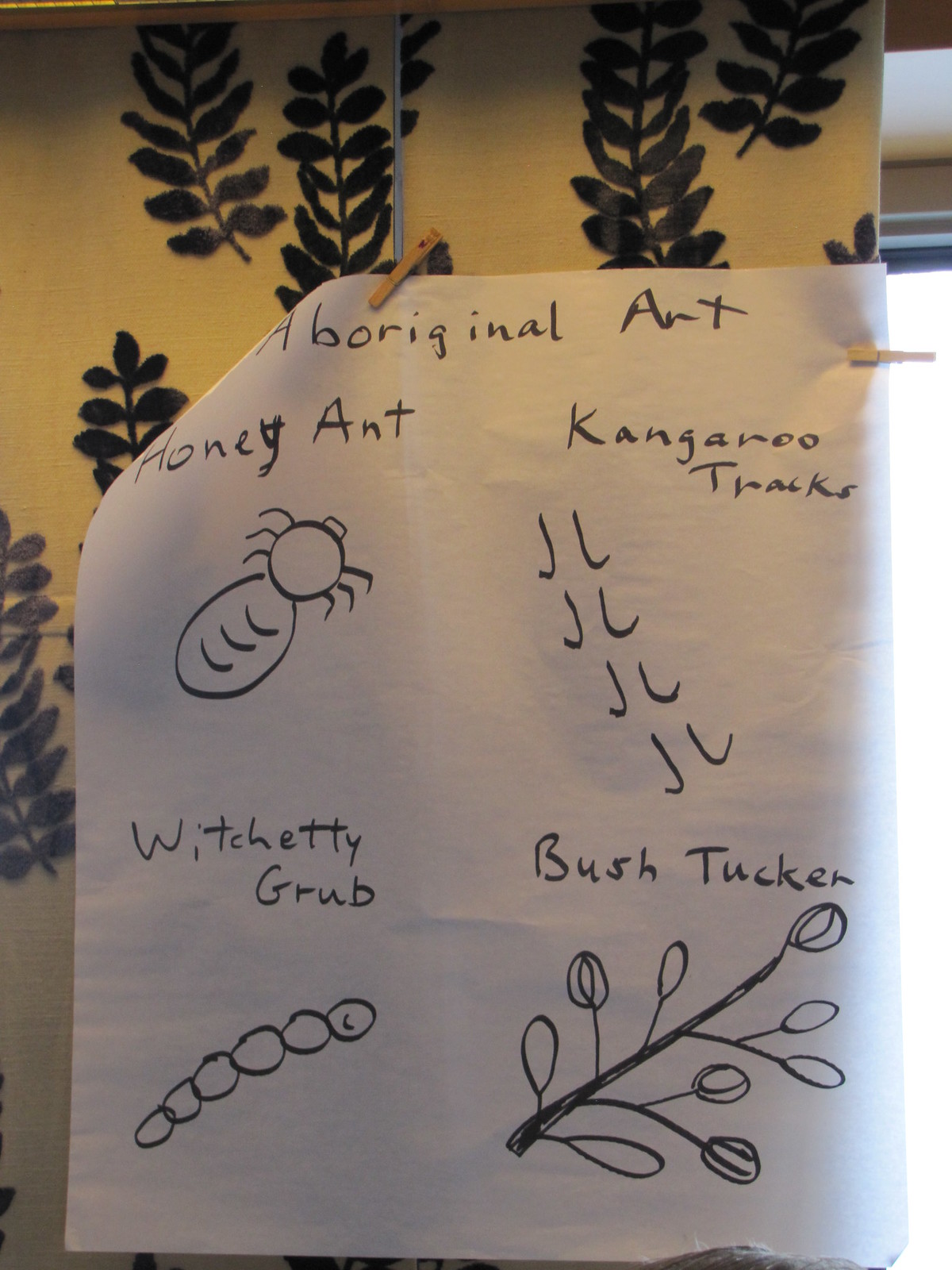The photograph captures a child-like depiction of Aboriginal art, featuring rudimentary sketches and natural elements. At the center of the image, a white piece of paper, secured by tan clothespins, displays black text and drawings labeled "Aboriginal art," "honey ant," "kangaroo tracks," "witchetty grub," and "bush tucker." The simple, almost crude illustrations resemble what a child might draw if asked to depict these subjects. The paper occupies the bottom three-fourths of the image. Behind this, the background wall is a yellow hue adorned with green decorative leaves, though it's unclear if the foliage is real or artificial. The overall scene conveys an innocent, youthful interpretation of Aboriginal themes, thoughtfully arranged with the sketches centrally positioned and the natural elements providing an intricate backdrop.